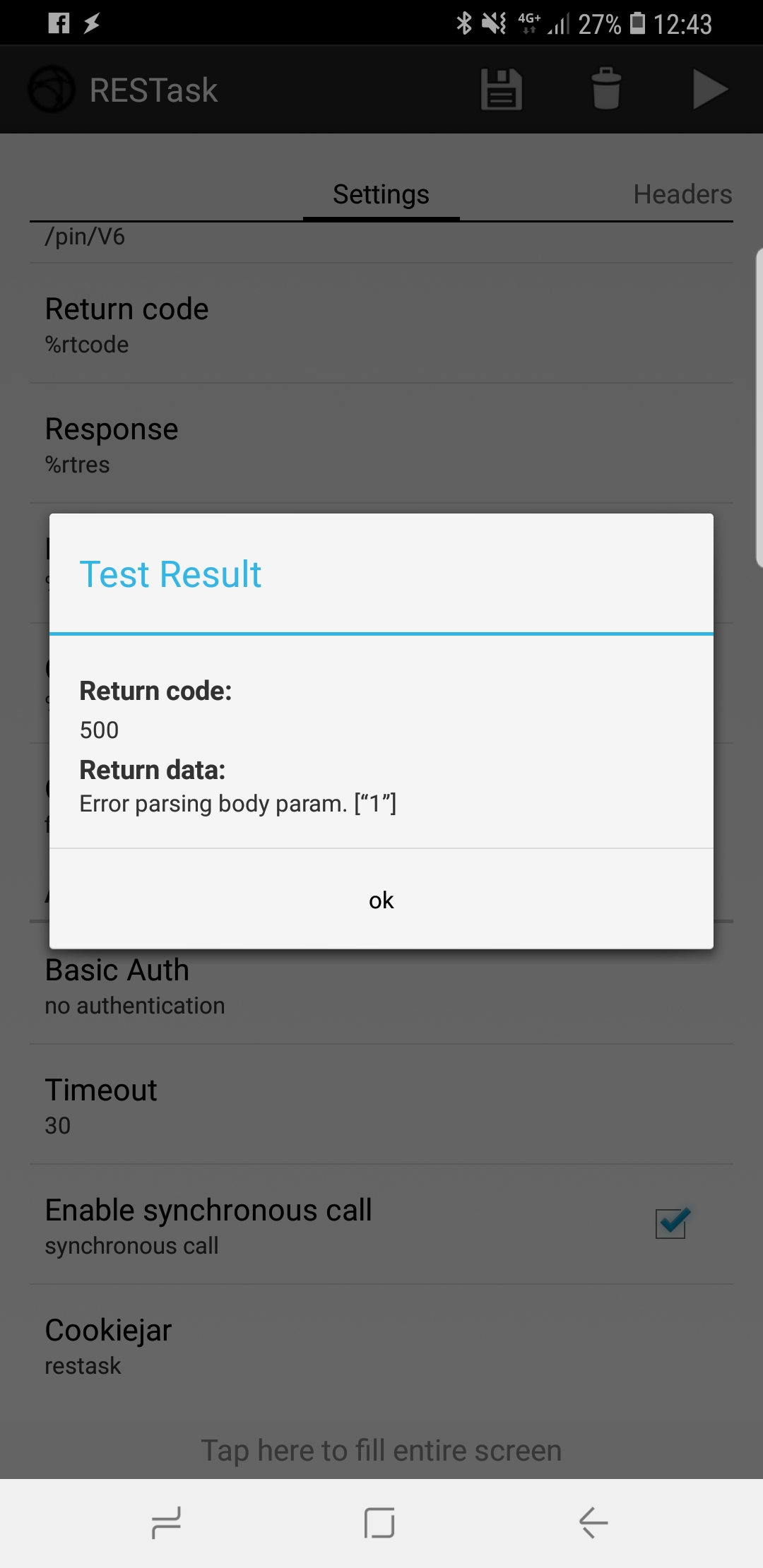The image is a screenshot taken from a mobile phone, with the device's status bar visible at the top. The time displayed is 12:43, positioned at the top right corner. Next to the time, a vertical battery symbol shows a charge level of 27%. Moving left, there is a phone signal strength icon displaying three out of four bars, followed by the label '4G+' indicating the network type. Further left, an audio icon that is crossed out signifies that audio is muted, and a Bluetooth icon indicates that Bluetooth is active.

On the top left side of the status bar, there are two more icons: the Facebook icon and a lightning symbol.

Central to the image is a squared box labeled "Test Result" at the top left, highlighted in blue. Below this label is a blue horizontal line. Within the box, two pieces of information are displayed. The first, "Return Code," is followed by the number 500. The second, "Return Data," is accompanied by the text "Error parsing body prim." At the bottom center of the box is a button labeled "OK."